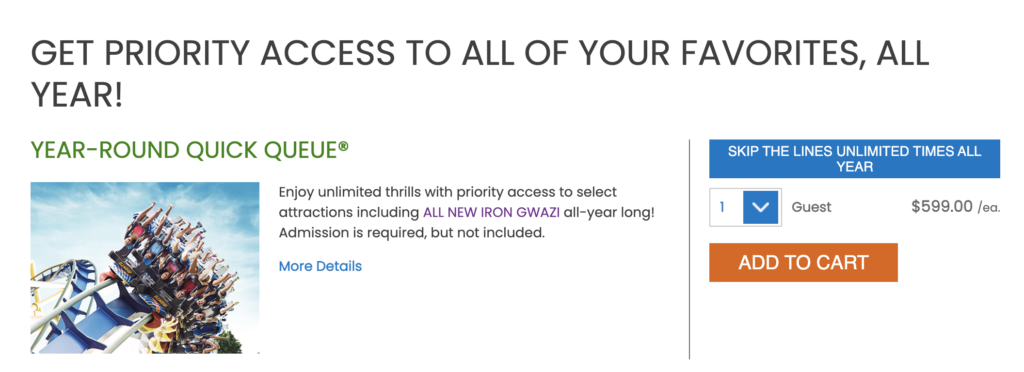**Caption:**

A web page presented in a clean, borderless rectangle showcases an enticing offer for thrill-seekers. The headline, boldly stating "GET PRIORITY ACCESS TO ALL OF YOUR FAVORITES, ALL YEAR!" in black text, stands out on a pristine white background. Below it, in green uppercase letters, the offer promises "YEAR-ROUND QUICK QUEUE™." 

The detailed description reads, "Enjoy unlimited thrills with priority access to selected attractions, including the all-new Iron Guazzis®," featuring "Iron Guazzis" prominently in purple. This is followed by, "all year long! Admission is required but not included." The phrase "for more details" is highlighted in blue to indicate a link.

To the right, an image captures the excitement of a roller coaster ride, with riders, some with arms raised high in exhilaration, seated across multiple rows. Adjacent to the image, the text promises, "Skip the line unlimited times all year," above a dropdown menu listing the price of $599.00 per guest. An orange "ADD TO CART" button invites immediate purchase.